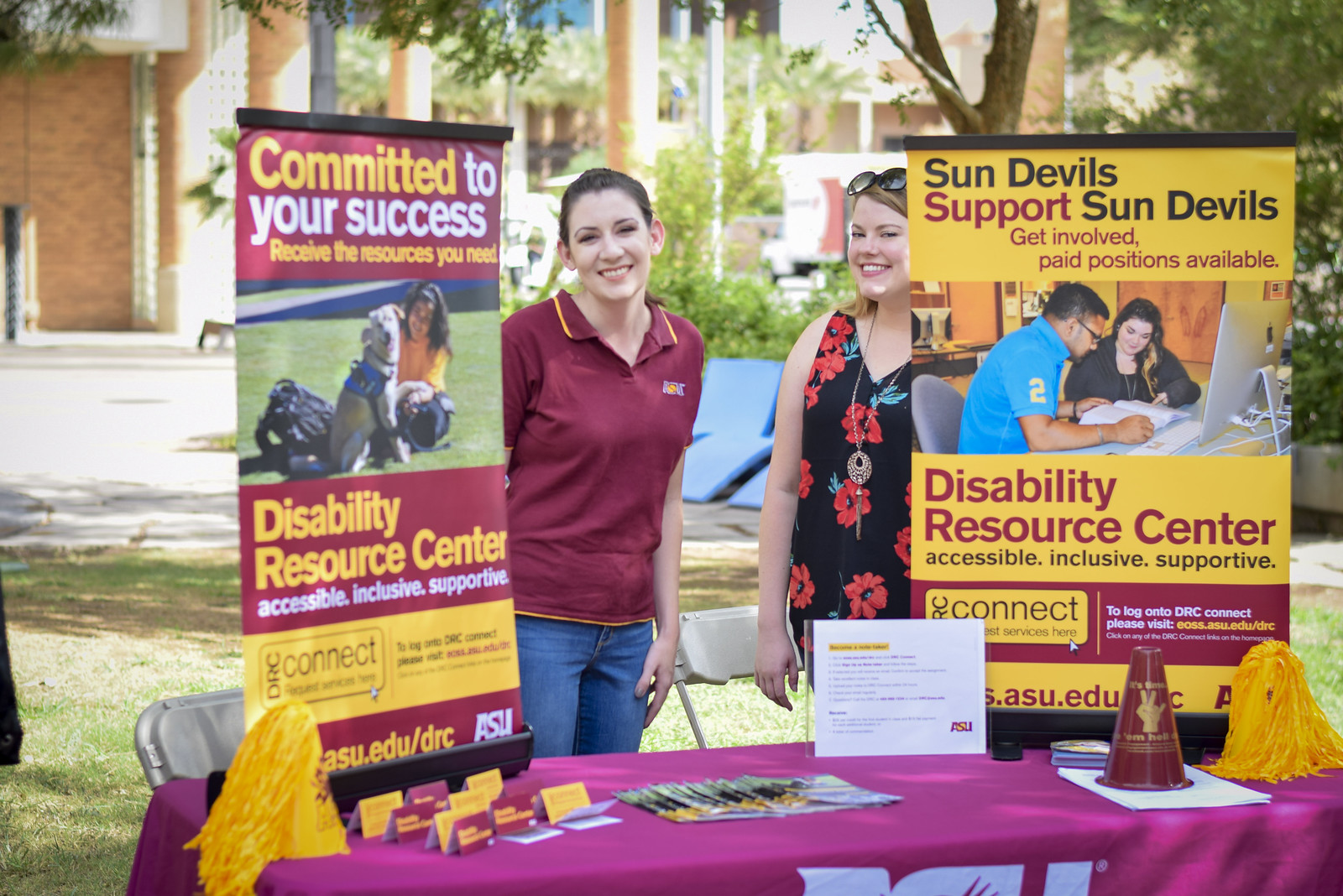In the photograph, two smiling women are situated at a table or booth, likely on a college campus. One woman, on the left, is wearing a maroon-colored, collared shirt accented with gold. To the left of her is a black-topped sign featuring the slogan, "Committed to your success," along with the text, "Receive the resources you need," followed by "Disability Resource Center: Accessible, inclusive, supportive," and further down, "DRC Connect." Adjacent to this sign is an image of a service dog and a woman.

Next to her on the right stands another woman in a black dress adorned with red flowers. Beside her is a yellow sign that reads, "Sun Devils support Sun Devils. Get involved. Paid positions available." The sign also includes the words "Disability Resource Center: Accessible, inclusive, supportive," and a picture of a woman at a laptop assisting someone. The table in front of them is scattered with flyers, business cards, and colorful pom-poms, adding to the lively atmosphere.